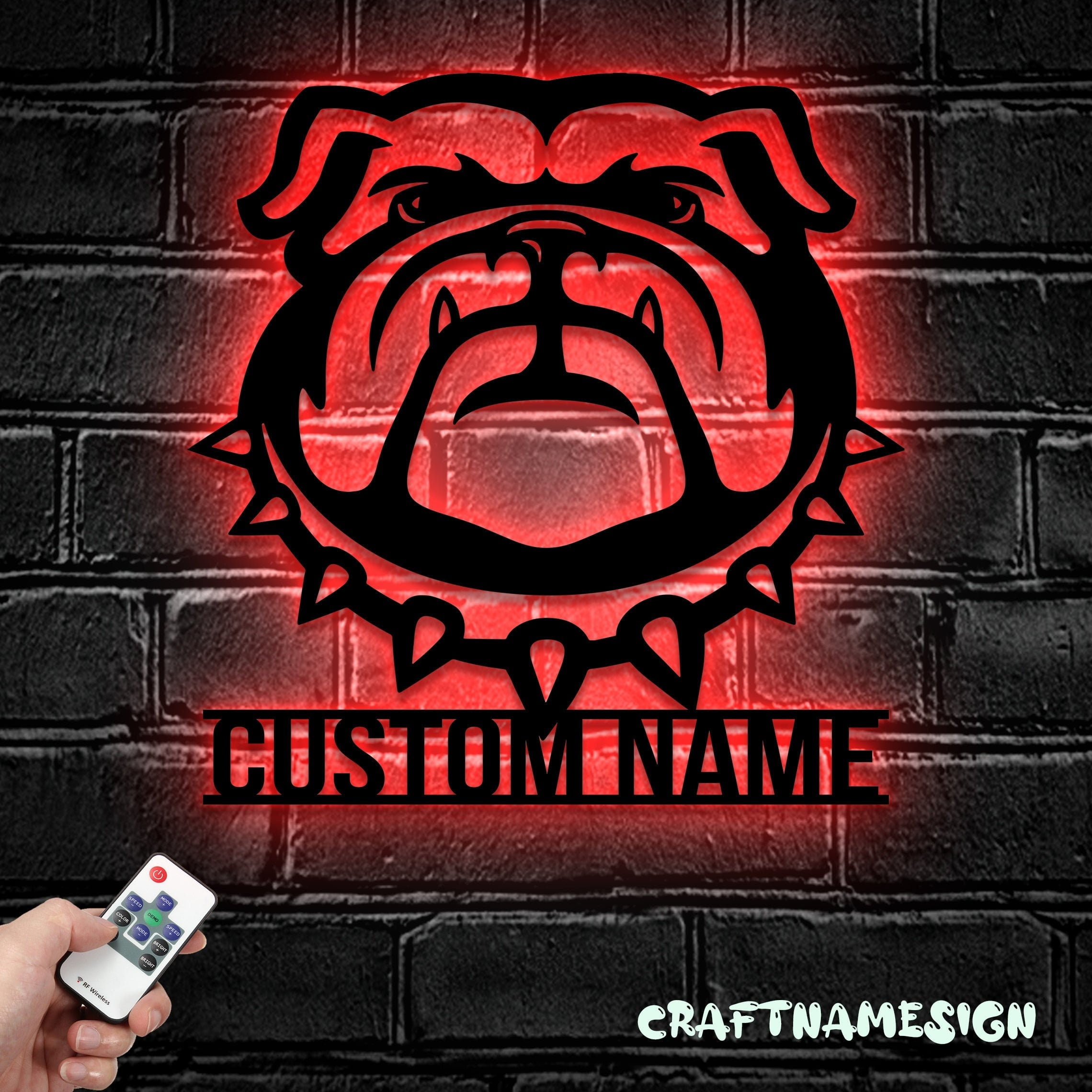In this colorful image, the backdrop is a black brick wall. Dominating the center is a stylized logo of a bulldog, outlined in thick black and designed to look like a neon sign, complete with an LED effect that gives off a red glow. The bulldog sports a spiked collar with two fangs protruding from its lower jaw. Below the bulldog, in all capital letters, is the phrase "CUSTOM NAME," signifying that customers can personalize the name beneath the bulldog image. Adding to the customization theme, the bulldog and text are illuminated from behind in red, enhancing the neon-like visual. In the lower left corner, a hand, likely belonging to a person of European descent, is visible, holding a white digital remote with blue, black, and red buttons. This hand suggests interaction or control over the digital projection. On the bottom right of the image, the words "craftnamesign" appear, written as a single concatenated word, possibly in a light teal or white color.